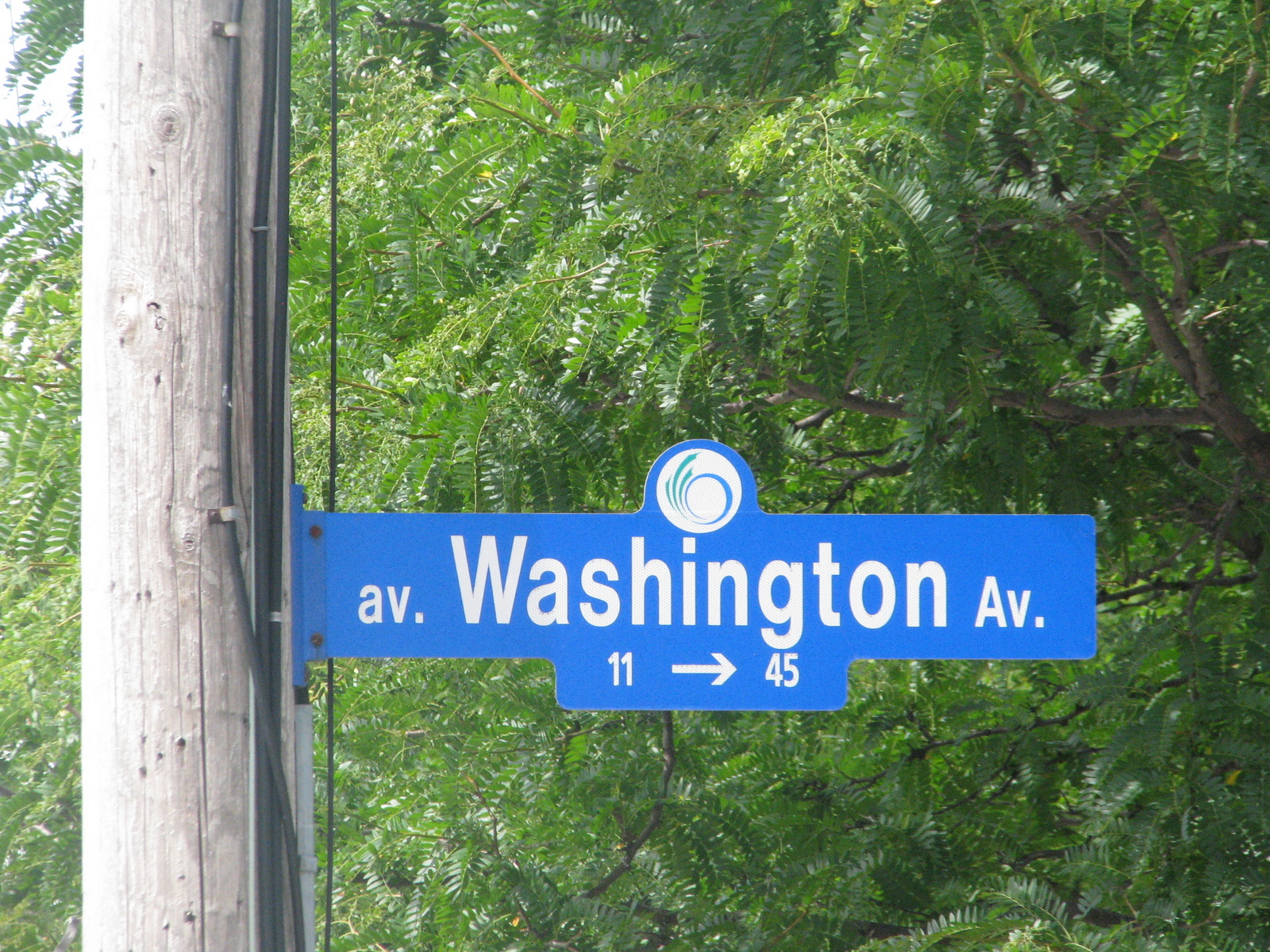This outdoor photograph captures a street sign mounted on a wooden pole, located to the left side of the image. Visible on the pole are several wires, likely cable lines, extending upwards. Behind the pole is a vibrant green tree with fern-like foliage, its branches gracefully drooping. The street sign itself is blue with white text. It features a distinct design with a white, bulbous section at the top, followed by a rectangular shape below. The sign prominently displays "AV.Washington AV." in white font, indicating Washington Avenue. Below the text, the numbers "11" and "45" are displayed, with an arrow pointing to the right located between them.